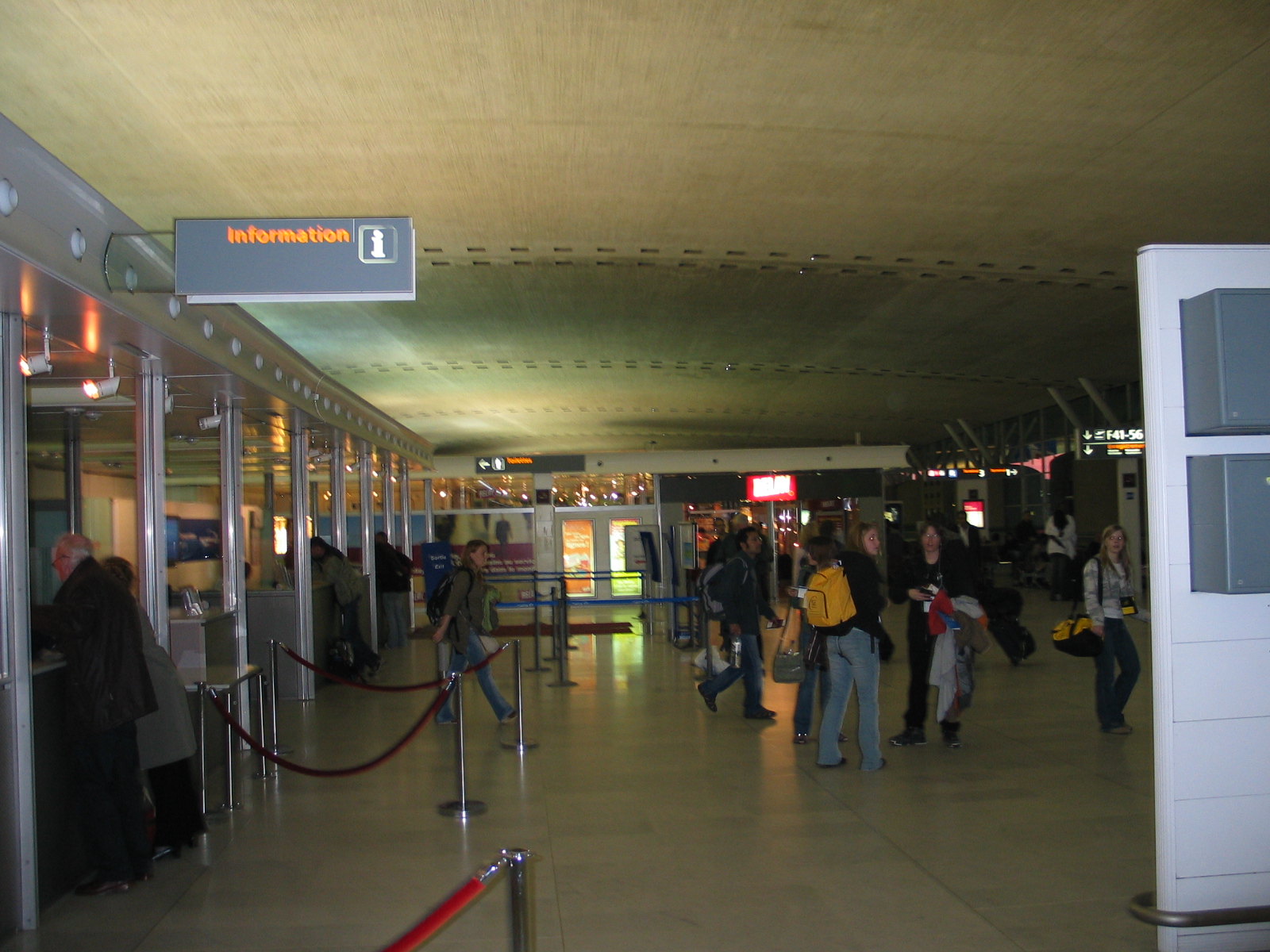The image depicts a bustling indoor terminal, likely a train station or airport, characterized by its relatively low lighting with illuminated sections in the distance. The foreground features a white wall adorned with metallic boxes and a concrete floor where numerous travelers, many carrying backpacks or luggage, navigate through the space. Prominently in the top left, an orange-lit "Information" sign marks an area composed of small booths where people are seen purchasing tickets from agents. Red rope barriers are positioned between metal poles, guiding the flow of the crowd. The reinforced concrete ceiling looms above, emphasizing the industrial feel of the environment. In the backdrop, a lit tunnel-like passage hints at the presence of stores or additional terminal areas, contributing to the overall lively and functional setting of this transportation hub.